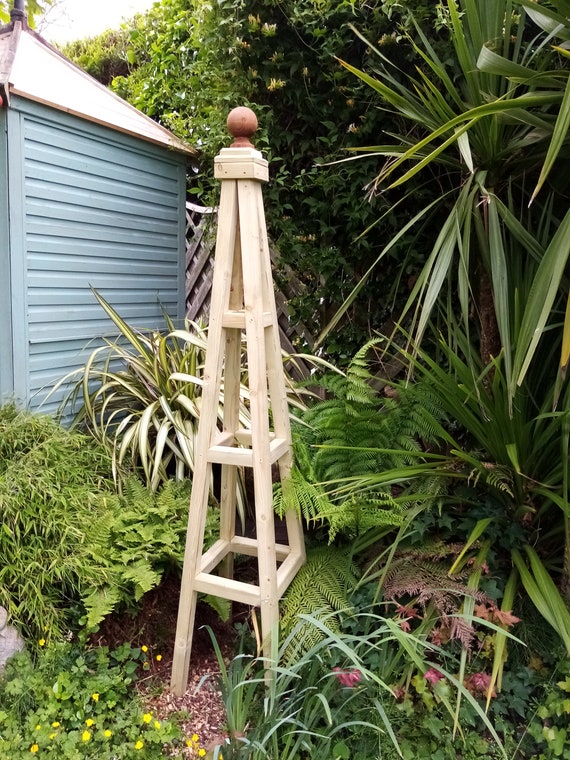The photograph captured outdoors during the daytime features a wooden tower prominently situated within a lush garden area. This rectangular image showcases the wooden tower, which is constructed from four wooden poles forming the corners of a square base, with three horizontal square rings connecting the poles. The structure extends upwards, culminating in a smaller square at the top, crowned with a small brown ball. Surrounding this wooden obelisk-like structure, the garden is vibrant with various plants and flowers. On the left and directly to the right, there are some sideways-growing leafy plants, and in the background, long single-blade leaves with white tops and green bottoms can be seen. In the bottom left corner, there are small green plants with yellow flowers, while pink flowers bloom on the right. The upper right corner of the image reveals a large banana tree. Adjacent to the wooden tower on the left side of the photograph, there is a blue shed with horizontal siding and a sloped, shiny roof. The background features a tree arching over the shed and a back fence further enhancing the garden's enclosed feel. Overall, the setting is bright, with daylight illuminating the scene, though the sky itself remains unseen beyond the bright light filtering through the greenery.